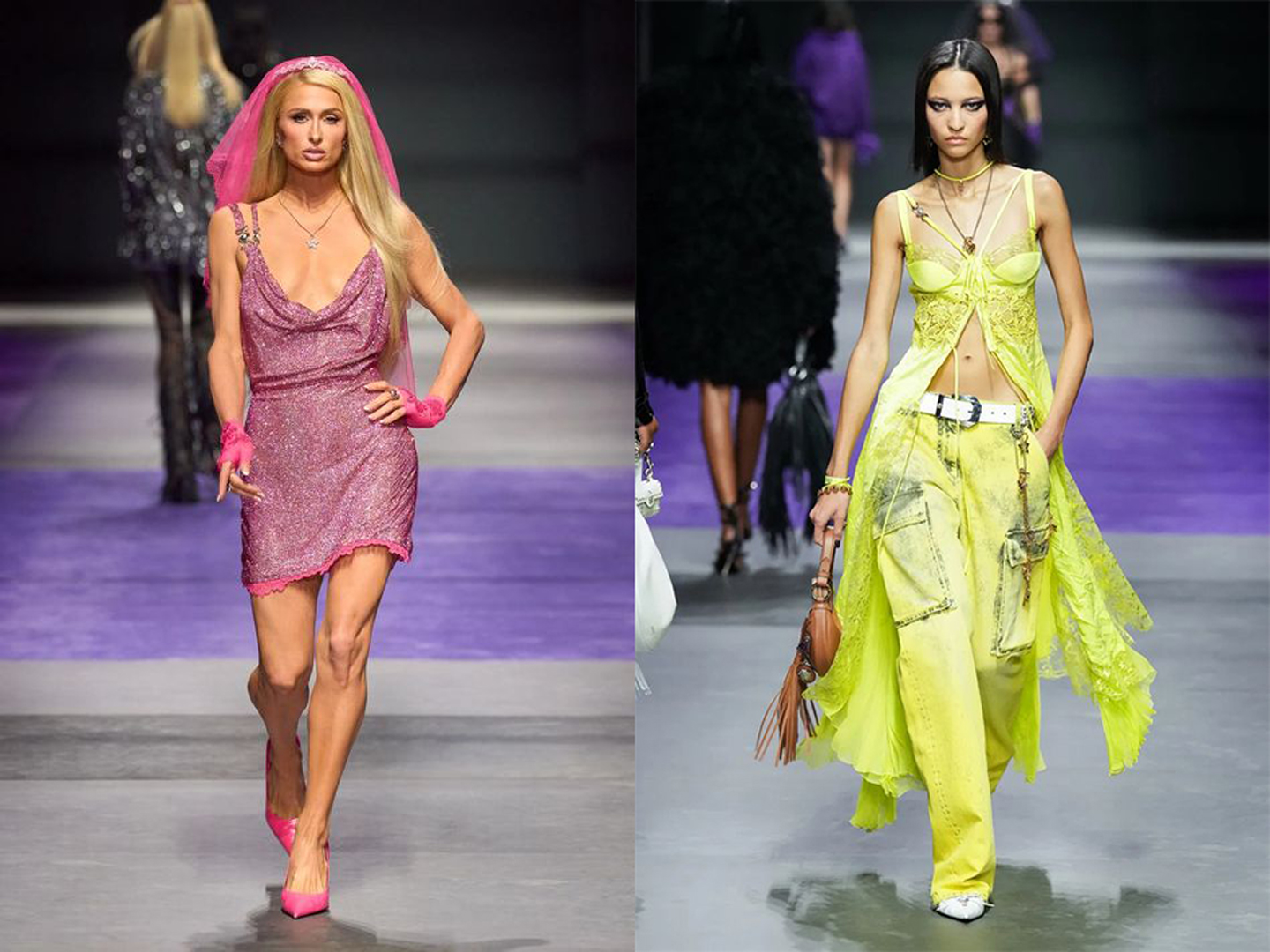The image features two fashion models walking down a gray runway accented with purple lines in a split-screen format. On the left is a model who closely resembles Paris Hilton, characterized by her long blonde hair and distinctive face. She is adorned in a shimmery pinkish-purple dress that is short, ending mid-thigh, and complemented by pink shoes and a pink veil. She also wears pink coverings on her wrists. On the right side is another model with long dark hair and bold black makeup. She sports a bright yellow outfit consisting of pants with oversized pockets outlined in dark blue and a skimpy top resembling a bra with a long, flowing train. She accessorizes with jewelry and holds a purse. Both images show additional models in the background walking down the runway. There is no text visible in the image.